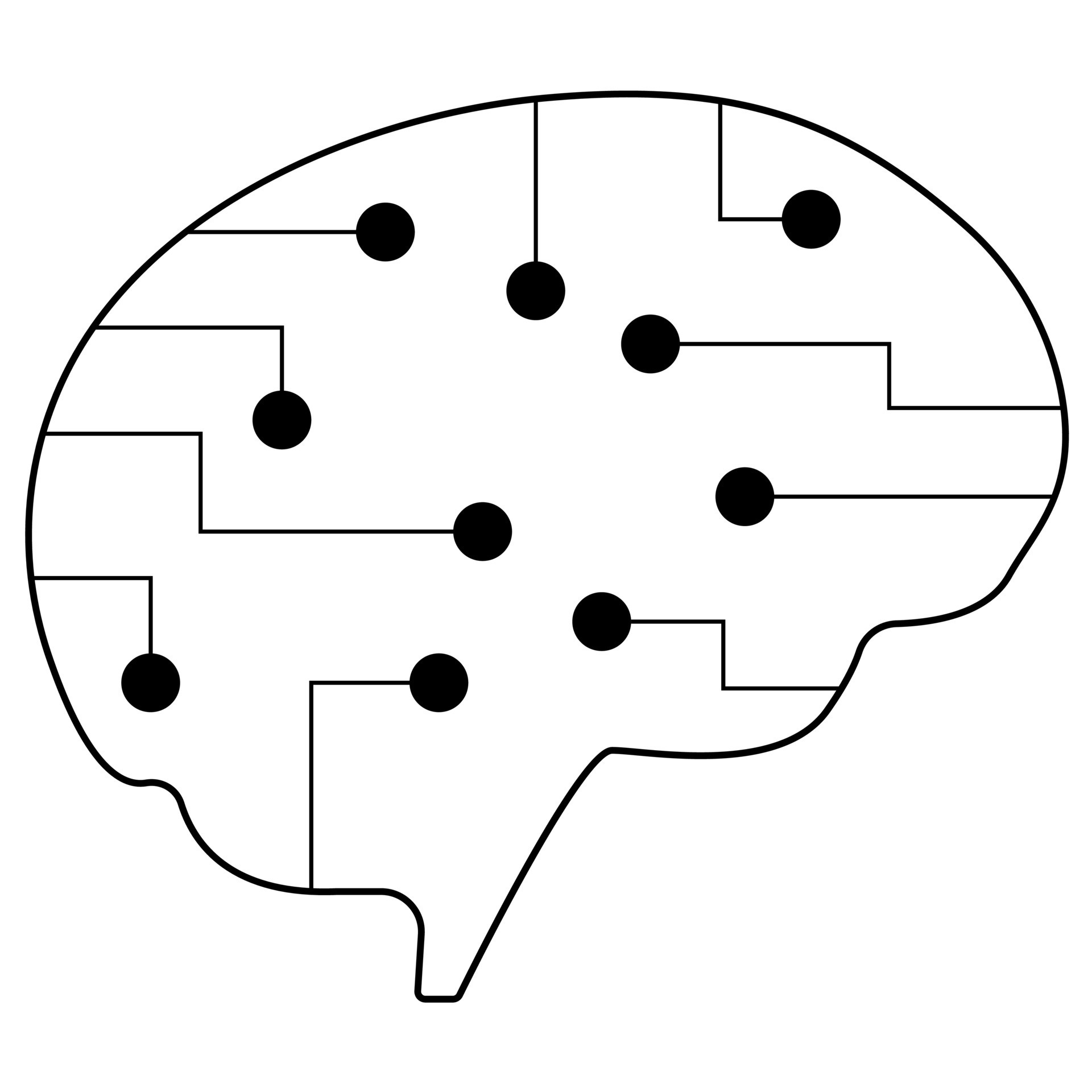The image is a simple, yet detailed, black line drawing resembling the shape of a brain. Its outline is formed by a medium-width black line that contours an abstract, brain-like shape, rounded at the top and dipping in undulating curves towards the sides and bottom. The entire drawing is set against a clean, white background with no additional text or identifiers. Inside this brain-shaped outline, there are nine distinct lines originating from various points along the outer edge, not touching each other and each terminating in a solid black circle or ball. These internal lines vary in direction and form sharp angles, bends, and zigzags. Among these, some lines jut out straight before turning down or right, while others make sharp turns. Notably, all the terminating black balls are directed either downwards or sideways, with none pointing upwards. The overall impression is that of an abstract, artistic rendition of a brain, accentuated by the stark contrast of black lines and circles against the white background.